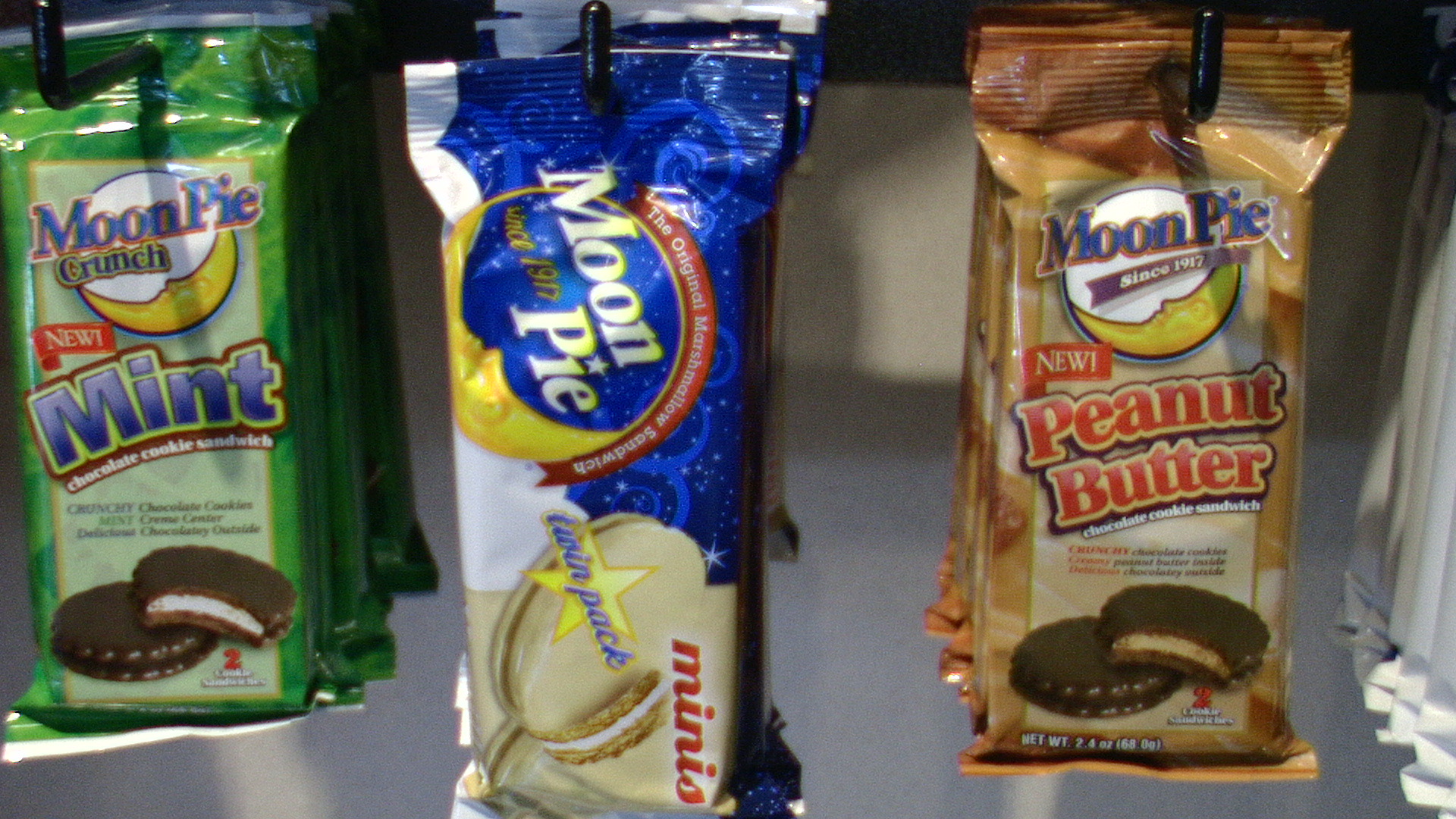Close-up image of three packaged desserts, displayed as if for sale in a convenience store. The leftmost package is green and prominently features the text "Moon Pie" in blue, with "Crunch" in yellow and blue, embossed on a yellow banana-like circle. Below, it states "new" in blue text and outlines "mint" in green. The description further reads "chocolate cookie sandwich," depicting dark brown chocolate cookies. The middle package shows "Moon Pie Minis" in a blue and white wrapper. To the right, there's another package marked with "Moon Pie" since 1917, highlighting "new peanut butter" in bright yellow text. This brown package showcases two brown cookies filled with a peanut butter filling. The background visible through the gaps between the packages is a neutral gray.